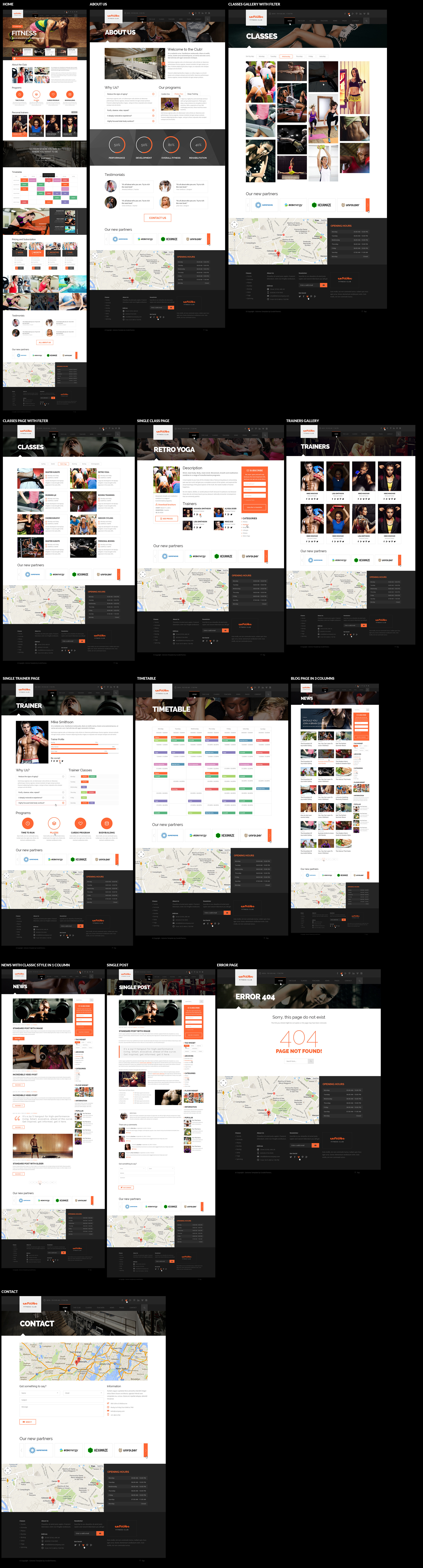The image features a predominantly black background decorated with numerous elements. Scattered throughout are various white and light gray rectangles, each containing indecipherable text and images. The majority of the white rectangles are layered over a slightly translucent map, except for the top three on the left-hand side which stand independently. Additionally, several orange rectangles are present within the composition. One notably large orange rectangle is centered amidst the images and encloses three horizontal white lines stacked vertically. Although there are smaller orange rectangles, discerning their details is challenging due to their size. The bottom section of the image prominently displays a comprehensive map, devoid of any accompanying pictures, with a solitary white rectangle situated just above it.